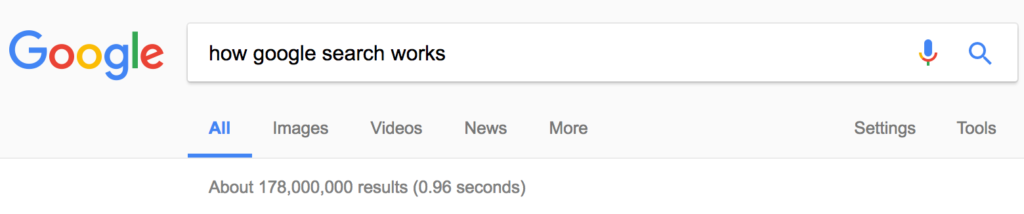A screenshot showcasing the Google search interface. The image is predominantly centered around the Google search bar, set against a softly shaded white-to-gray gradient background running horizontally across the frame. This gradient encompasses the vibrant, multi-colored Google logo situated on the upper left side of the image with each character colored distinctly – blue 'G', red 'O', yellow 'O', blue 'G', green 'L', and red 'E'. Below the logo, the search bar prominently displays the query “how Google search works.” Beneath the search bar is a menu bar, which eventually transitions to plain white. Below this menu bar, in grayish font, is a brief note indicating the number of search results, "About 178 million results (0.96 seconds)."